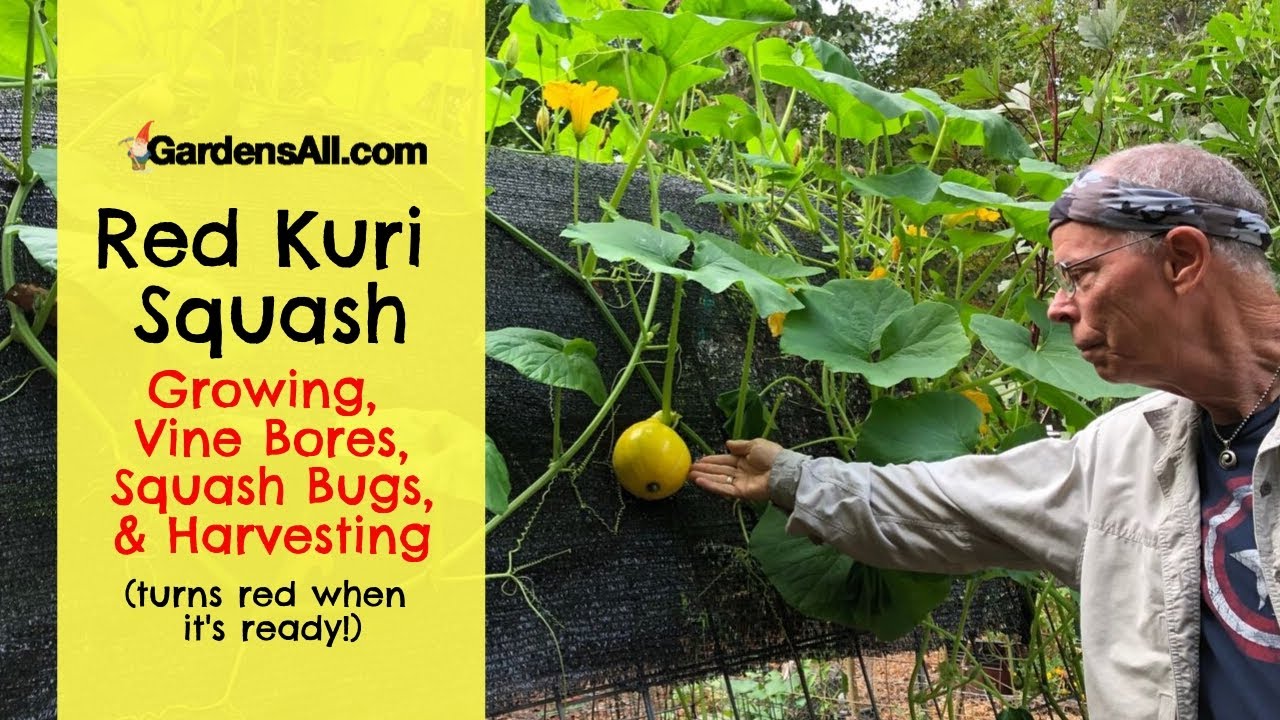Title Graphic for GardensAll.com Article: "Red Curry Squash - Growing Vine Bores, Squash Bugs, and Harvesting"

The image features a title graphic for GardensAll.com with the article title prominently displayed: "Red Curry Squash - Growing Vine Bores, Squash Bugs, and Harvesting" followed by a note in parentheses indicating that the squash "turns red when it's ready." The scene includes a yellow billboard-style element typical in the magazine world.

Adjacent to the title graphic, a man is captured reaching out to touch one of the Red Curry Squash, which is currently yellow. He is dressed in a red shirt, white jacket, and a headband. The squash vines are visibly growing tall, extending high above the ground, adorned with large yellow blossoms. Below, other plants thrive, bordered by a stone or brick wall that provides a rustic backdrop to the lush growth.